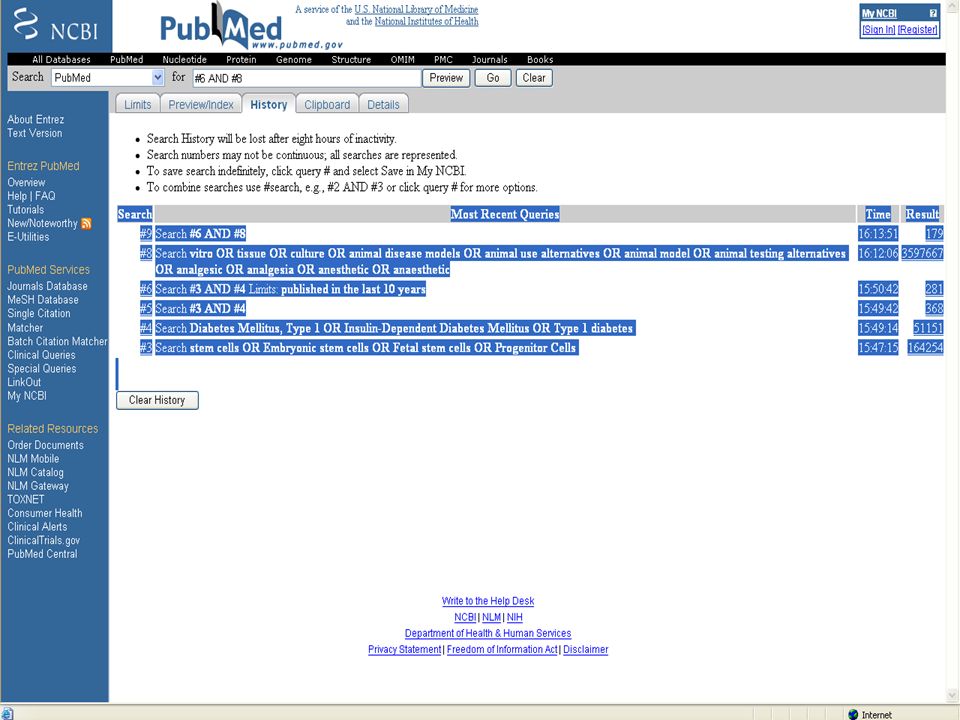This detailed and cleaned-up caption could be used to describe the image:

The image showcases a web page dedicated to medical publications, sponsored by the National Center for Biotechnology Information (NCBI). The color scheme of the page is primarily blue, gray, and white. Positioned at the top left, the NCBI logo features a spiral resembling the symbol of the Hippocratic Oath. The website is identified as PubMed, accessible via PubMed.gov, and is a part of the U.S. National Library of Medicine.

The interface includes functionalities allowing users to create and manage their accounts, as indicated by the “Identify My NCBI” section on the right. The central feature is a basic search engine where users can look for various types of medical documents. The search results page provides additional options such as "Limits," "Preview/Index," "History," "Clipboard," and "Details," which help refine and manage search queries.

An important notice warns users that search history will be lost after eight hours of inactivity, emphasizing that search numbers may not be continuous but all searches are logged. Users have the option to save searches indefinitely by clicking the provided query links. Recent search queries, such as for diabetes and animal diseases, are listed with timestamps and results indicating the number of articles found.

On the left side, navigation options are available under sections like PubMed Services and Resources. At the bottom, several clickable links lead to different services, including a help desk and various health-related web pages, providing additional support and information.